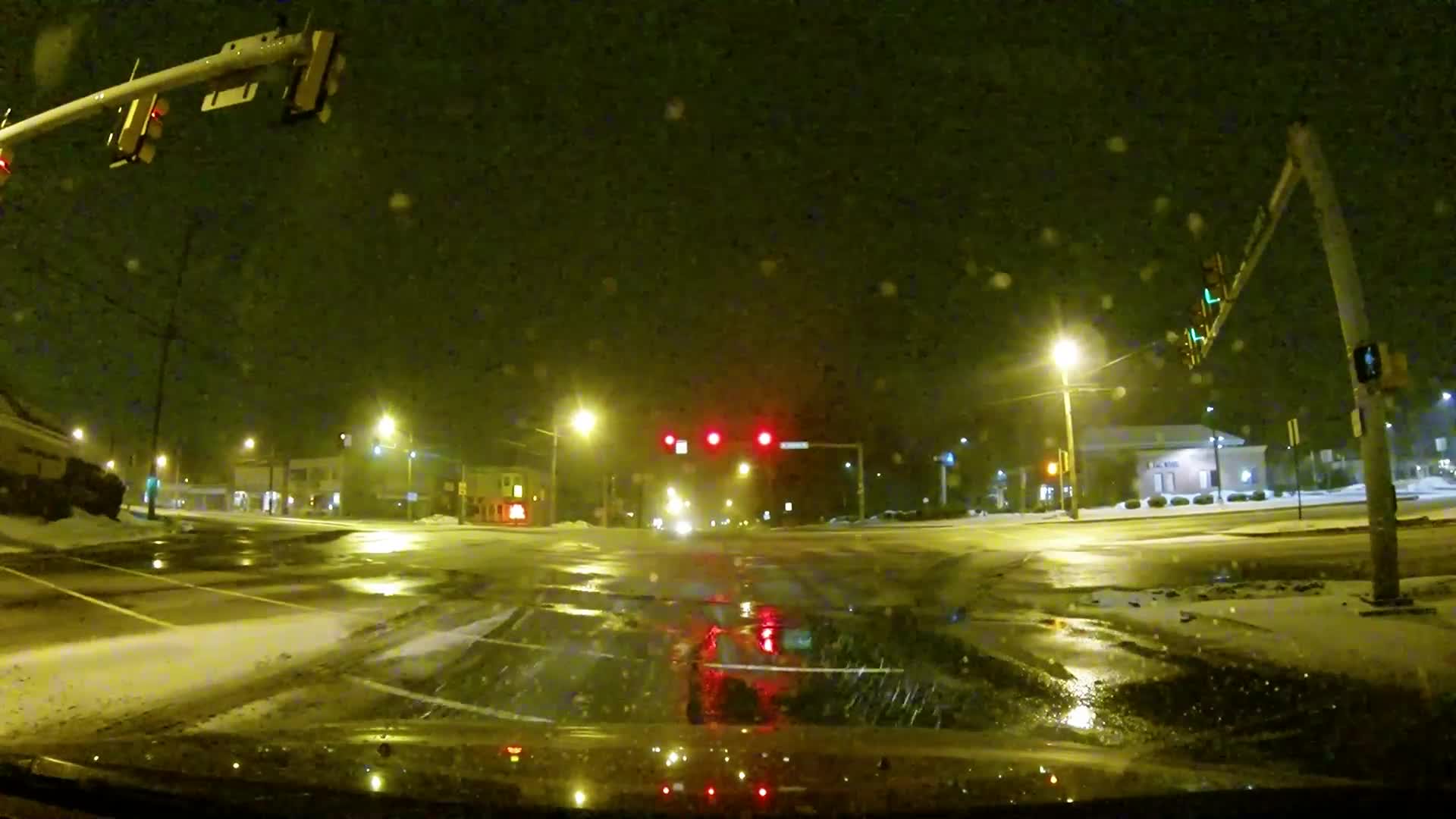This photograph, taken from the perspective of a vehicle through its windshield, captures the essence of a dark, rainy night. The hood of the vehicle, a light color, is partially visible, streaked with raindrops and reflecting splashes of water. The ground below glistens with moisture, evidence of the continuous downpour. In the distance, a streetlight casts a faint glow over the intersection ahead. Three red traffic lights are aligned horizontally, punctuating the night with their glow. To the upper left of the intersection, an office building looms subtly in the shadows, while to the right, a one-story structure, possibly a bank, stands quietly. The scene is illuminated primarily by the streetlights and the vehicle's headlights, creating a hauntingly serene yet vivid depiction of a rainy night in the city.